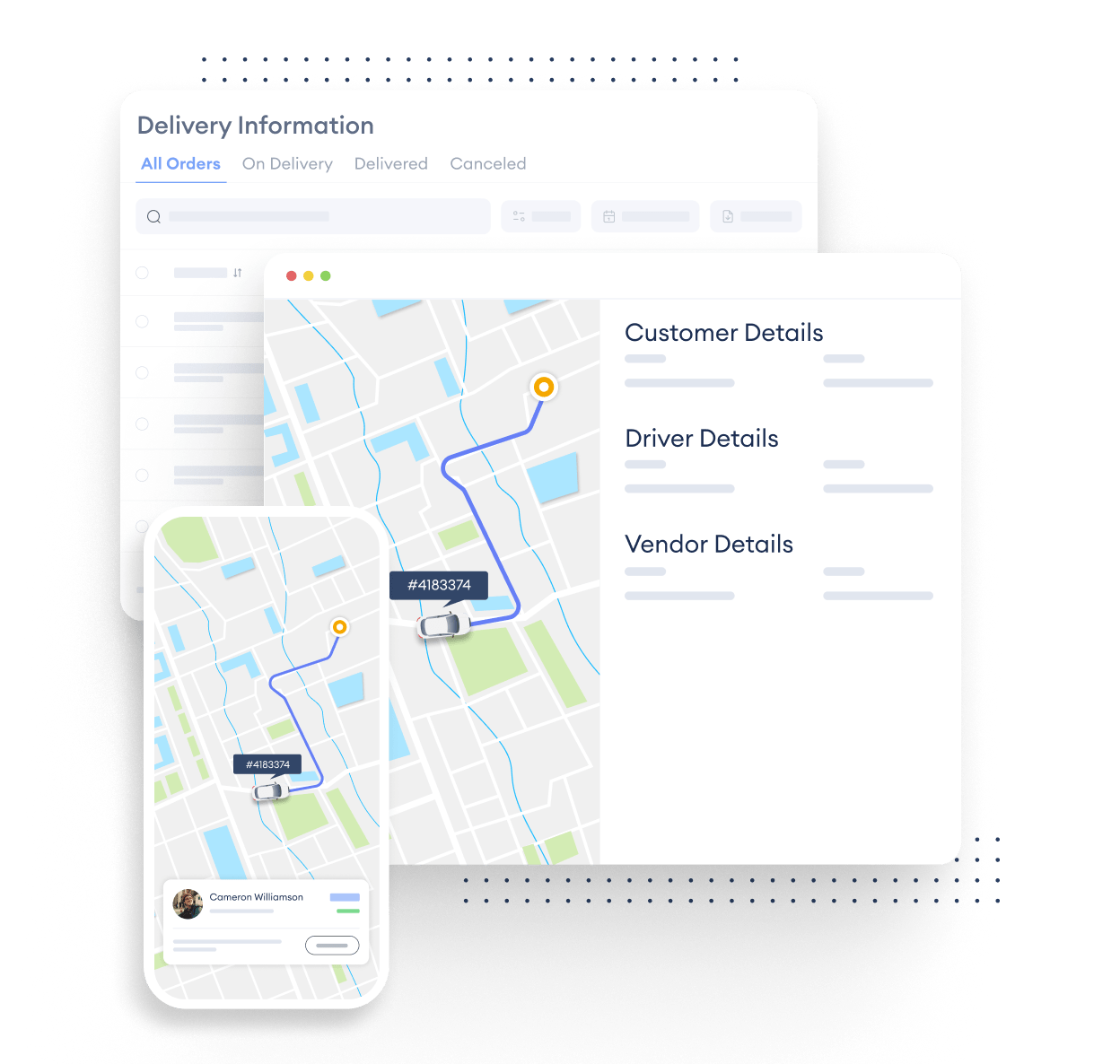The image depicts a detailed delivery information interface. At the top, in blue blocks, there is a hashtag symbol followed by the number 4183374. Below this identifier, the main section shows a map illustrating a car's journey, with a blue line tracing the vehicle's route. This line navigates through various roads, land masses, and bodies of water, eventually ending at a circle with a yellow center, likely indicating the final destination.

To the left of the image, the interface indicates it is being viewed on a desktop, with a smaller inset at the bottom left showing a similar interface on a mobile device. The top left corner prominently shows the label "Delivery Information," with several tabs for filtering orders: "All Orders," "On Delivery," "Delivered," and "Canceled." To the right, there are sections titled "Customer Details," "Driver Details," and "Vendor Details," though the specific entries within these sections are obscured for privacy.

In summary, the image provides a comprehensive overview of the delivery process, combining route visualization with detailed tabs for managing orders and user information, all within a dual-platform interface visible on both desktop and mobile devices.